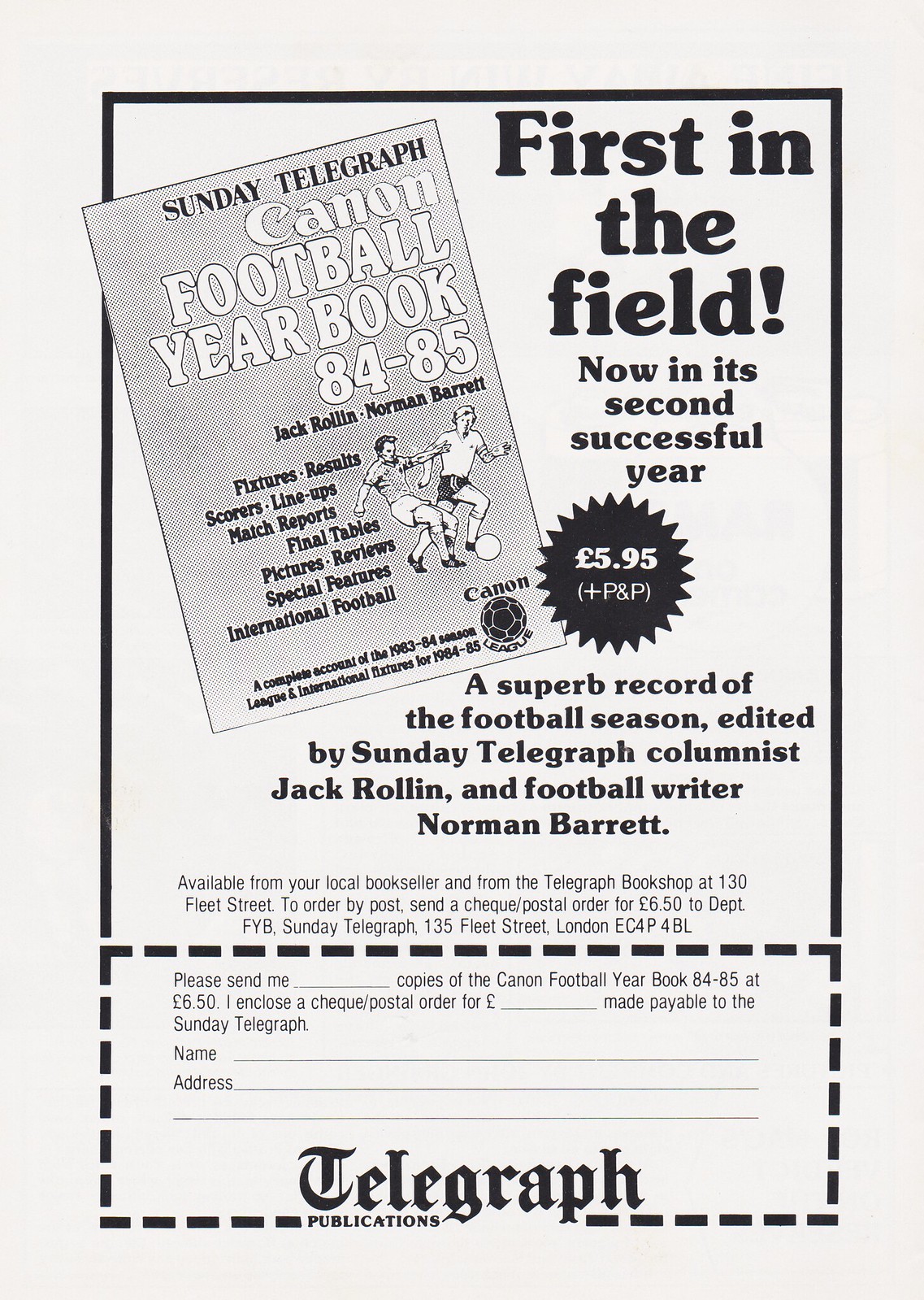This image is an advertisement in a pamphlet, promoting the "Canon Football Yearbook" for the 1984-85 football season. The background has a slightly pinkish off-white hue with a black border. Displayed prominently in black text, the ad reads: "First in the field! Now in its second successful year," followed by the price, "£5.95 P&P." The ad highlights the yearbook as "A superb record of the football season," edited by Sunday Telegraph columnist Jack Rollin and football writer Norman Barrett. The pamphlet includes an illustration of the yearbook cover, featuring two football players in action. The illustration notes the contents such as fixtures, results, scores, lineups, match reports, final tables, pictures, reviews, special features, and international football. Below the main text, there's a perforated order form for readers to fill in their details and purchase the yearbook.